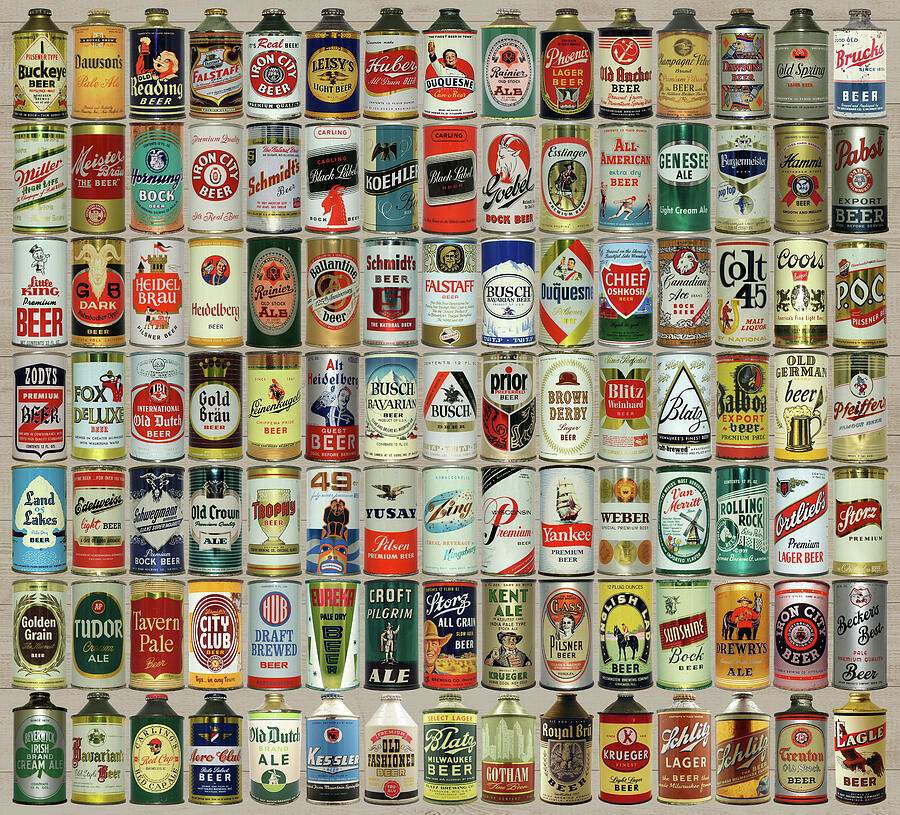The image showcases a meticulously arranged collection of vintage beer cans, organized in a grid of 15 columns and 7 rows, totaling 105 cans. These cans, dating back many years, reflect the evolution of beer container design. Predominantly tin, most cans lack modern pull tabs, indicating they were opened with a can opener or by popping the top. The collection features a colorful array of labels from various brands, such as Buckeye, Union City, Iron City, Colt 45, Coors, Bush, Trophy, Kent Ale, Kruger, Tudor, Golden Grain, and Land O' Lakes, with prominent colors including shades of red, white, gold, and silver. Some cans have a straight, cylindrical shape reminiscent of oil canisters, while others have angled tops akin to stout bottles with twist caps. All labels are uniformly positioned to face forward, showcasing the diverse heritage of beer branding and packaging.